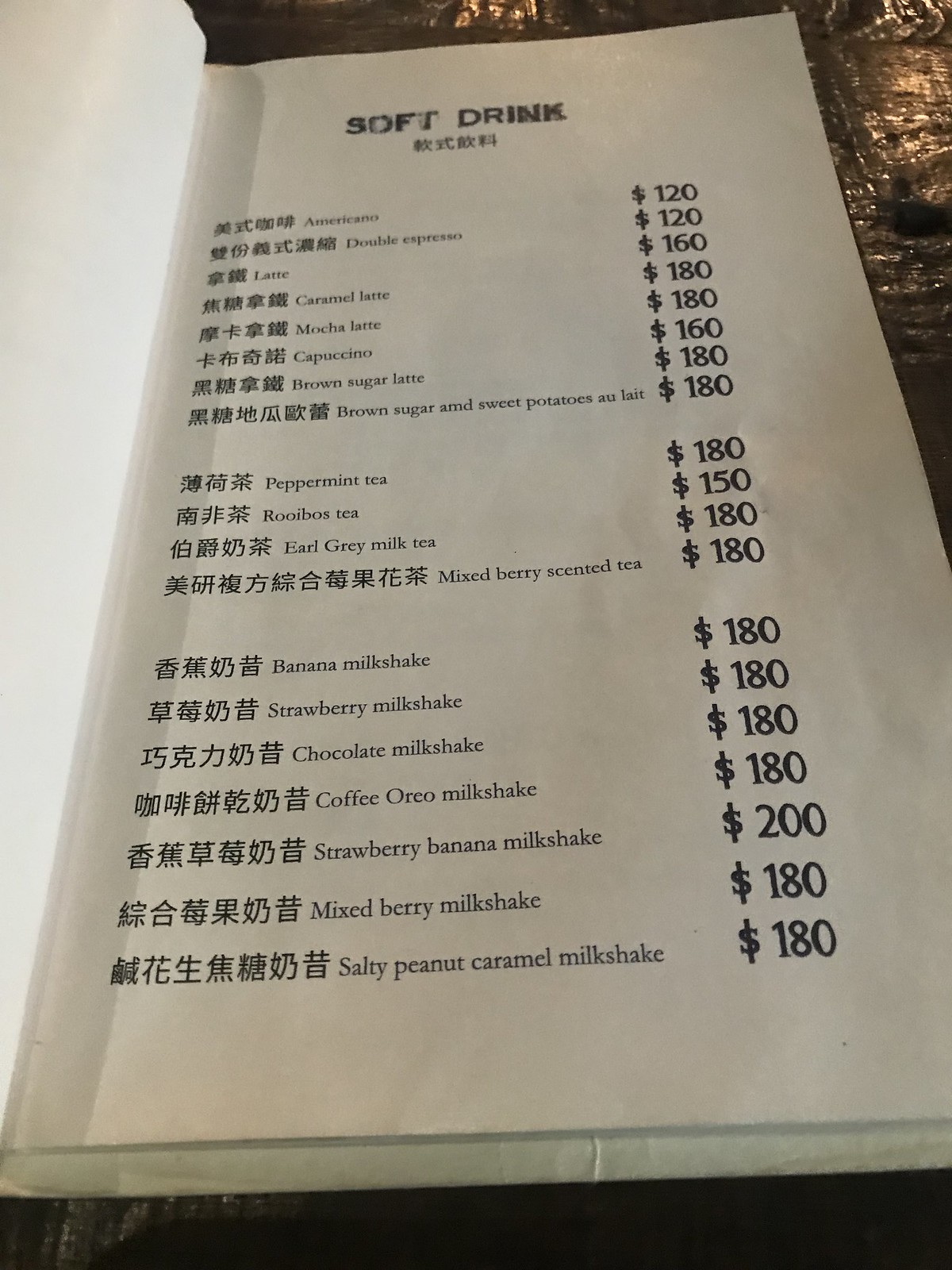This image captures an open menu displaying a variety of beverages written in English and Chinese characters. The title "SOFT DRINK" is prominently shown at the top in bold, uppercase black font. Below, the menu lists an array of drinks with their respective prices in dollars alongside each item:

- Americano: $120
- Double Espresso: $120
- Latte: $160
- Caramel Latte: $180
- Mocha Latte: $180
- Cappuccino: $160
- Brown Sugar Latte: $180
- Brown Sugar and Sweet Potatoes: $180
- Peppermint Tea: $180
- Rooibos Tea: $150
- Earl Grey Milk Tea: $180
- Mixed Berry Scented Tea: $180
- Banana Milkshake: $180
- Strawberry Milkshake: $180
- Chocolate Milkshake: $180
- Coffee Oreo Milkshake: $180
- Strawberry Banana Milkshake: $200
- Mixed Berry Milkshake: $180
- Salty Peanut Caramel Milkshake: $180